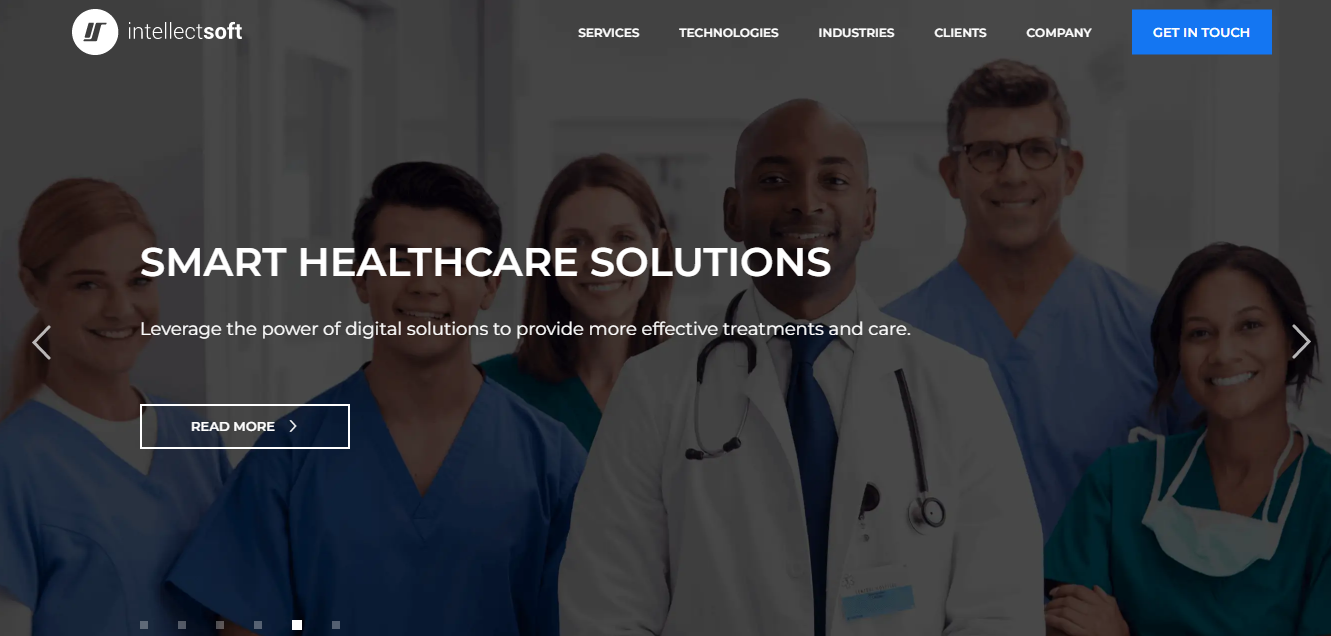This screenshot captures the home page of a website belonging to IntellectSoft, a company specializing in digital solutions for healthcare. The page is dominated by a large, slightly dimmed photograph that serves as a background, giving it a grayish tint. Superimposed on the image, in bold white font, are the words "Smart Health Care Solutions," with a subheading that reads, "Leverage the power of digital solutions to provide more effective treatments and care."

In the upper left-hand corner of the page, the company name "IntellectSoft" is displayed as a single word, with "Soft" in bold font. Next to the company name is a stylized logo featuring the letters "I" and "S" within a circle, rendered in a darker font. 

The navigation menu appears in white text and includes the options: Services, Technologies, Industries, Clients, and Company. In the upper right-hand corner, there is a blue rectangle with the white text "Get in Touch."

The background photograph showcases several healthcare professionals. On the right side, there is a black male doctor wearing a white coat and a stethoscope. To his left is a white male surgeon dressed in blue surgical scrubs, and next to him is a light-skinned black female healthcare professional in green surgical scrubs, with a surgical mask hanging around her neck. On the left side of the image, there are three more individuals: a white female healthcare worker in light blue scrubs, an Asian male in blue scrubs, and another white female in green scrubs. 

The overall design integrates the visuals and text seamlessly, highlighting IntellectSoft's commitment to innovative digital solutions in healthcare.